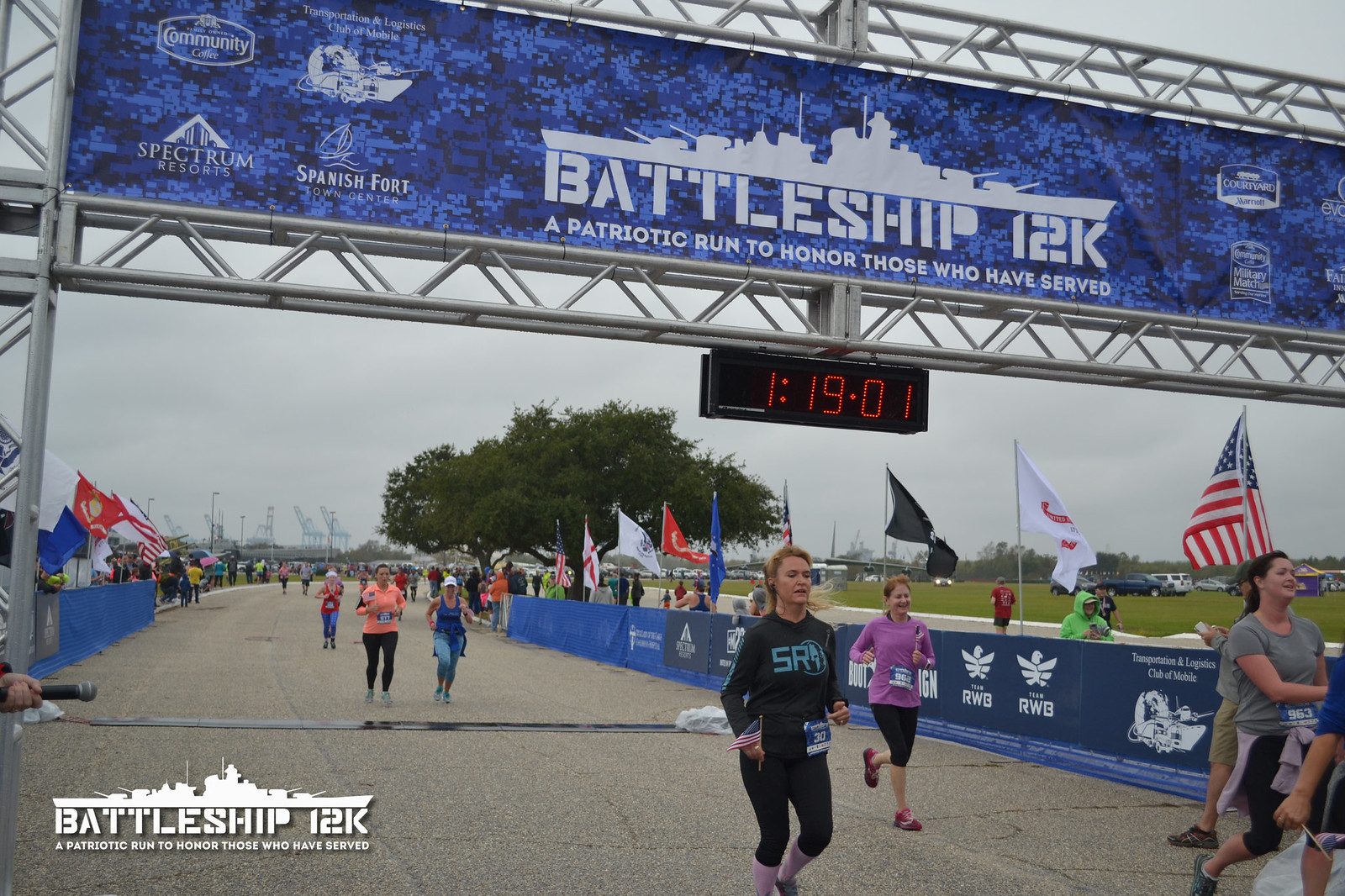The photograph captures the finish line of the Spectrum Resorts Spanish Fort Battleship 12K, a patriotic run to honor those who have served. The scene is set outdoors during the daytime, depicting a group of runners, primarily middle-aged women, crossing the finish line on a gray paved area flanked by low walls adorned with blue-bordered advertisements. A prominent metal framework stretches from left to right above the runners, supporting a blue banner with white print, featuring a white silhouette of an old battleship and the text: "Battleship 12K, a patriotic run to honor those who have served." Below the banner hangs a black digital clock displaying the time 1:19:01 in red digits. To the right of the track, a line of flags, including an American flag prominently near the viewer, adds a patriotic touch. In the backdrop, a wide, bushy tree provides a natural contrast to the structured elements. The lower left corner of the photograph features another small white outline of a battleship with the event’s title, reinforcing the theme. The background merges into a gray sky, completing the scene.